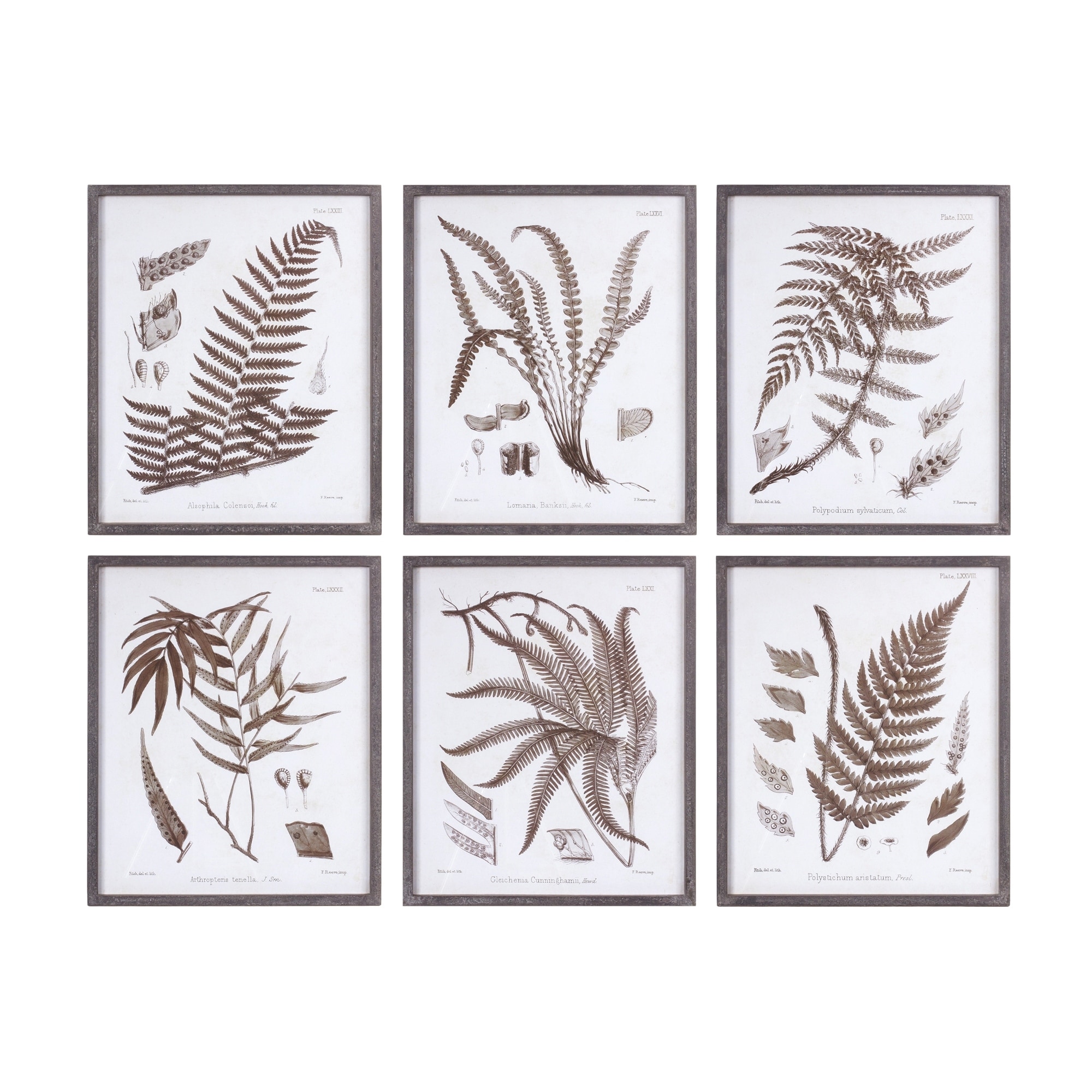The image is a detailed composition of six framed photographs arranged in two rows of three, each positioned tightly next to each other. The overall layout is landscape, although each individual frame is in portrait orientation. The frames are a uniform grayish wooden color, matching the hue of the leaves depicted within them, creating a cohesive and elegant appearance. Each frame showcases different leaves with various shapes and patterns, such as one resembling a sailboat and another in the shape of a V, while other leaves have more random shapes and patterns, possibly resembling wheat or grain.

The backdrop of the images is a clean white, enhancing the uniformity and minimalistic aesthetic. Small, unreadable text is placed both at the top right corner, possibly indicating dates, and at the bottom of each frame, likely providing descriptions of the leaf types. Despite the unreadable text, the images convey a sense of botanical diversity and study, as if part of a larger educational set. Each frame seems to focus on a particular leaf or branch, presenting both an overall view and a detailed close-up within the same frame.